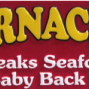This is a close-up image of a very small section of a larger sign, approximately two inches by two inches, with a plain red background. Dominating the upper portion of the image are large, thick yellow letters that read "R-N-A-C." These letters are cut off and seem to be part of a larger word. Below this, there are two lines of smaller white text; the first line reads "E-A-K-S," which, combined with the partially visible letters next to it, likely forms "STEAKS" or "SEAFOOD." The second line contains the letters "A-B-Y" followed by the word "BACK," suggesting it could be part of "BABY BACK." The imagery and text alignment make it evident that this is a cropped section of a sign advertising food items, but the fragmentary nature obscures the complete message.